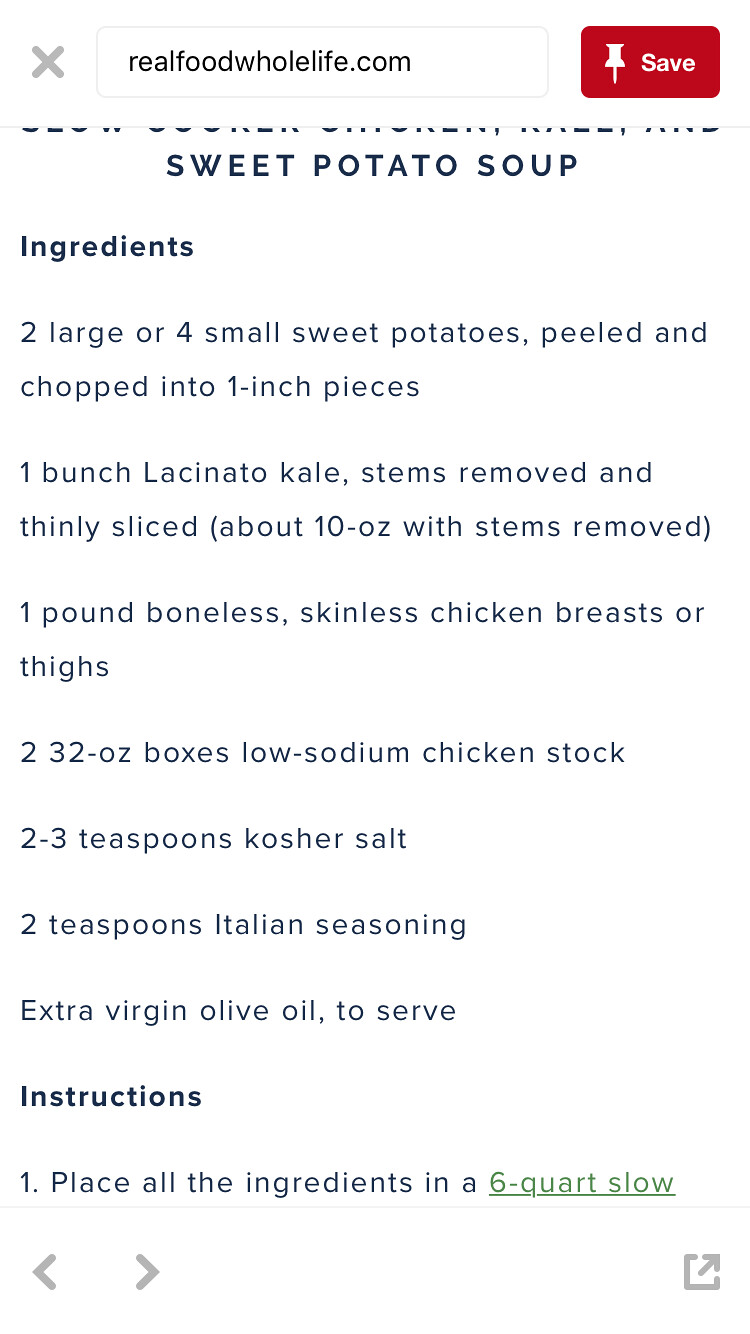This is a detailed image of a sweet potato soup recipe from Pinterest. At the top of the image, within a small rectangle, the web address "realfoodwholelife.com" is prominently displayed in black letters on a white background. Adjacent to it is a red rectangle featuring a save button, complete with a thumbtack icon. Beneath the search bar, which also has an 'X' to the left indicating it could be cleared, the title of the recipe, "Sweet Potato Soup," is clearly visible.

The ingredients are listed left-justified and include: two large or four small sweet potatoes (peeled and chopped into one-inch pieces), one bunch of lacinato kale (stems removed and thinly sliced, approximately ten ounces without stems), one pound of boneless, skinless chicken breasts or thighs, two 32-ounce boxes of low sodium chicken stock, two to three teaspoons of kosher salt, two teaspoons of Italian seasoning, and extra virgin olive oil to serve.

Instructions begin with the first step: "Place all the ingredients in a six-quart slow..." but the text is cut off there. Navigation arrows within the image indicate options to go back or forward a page.